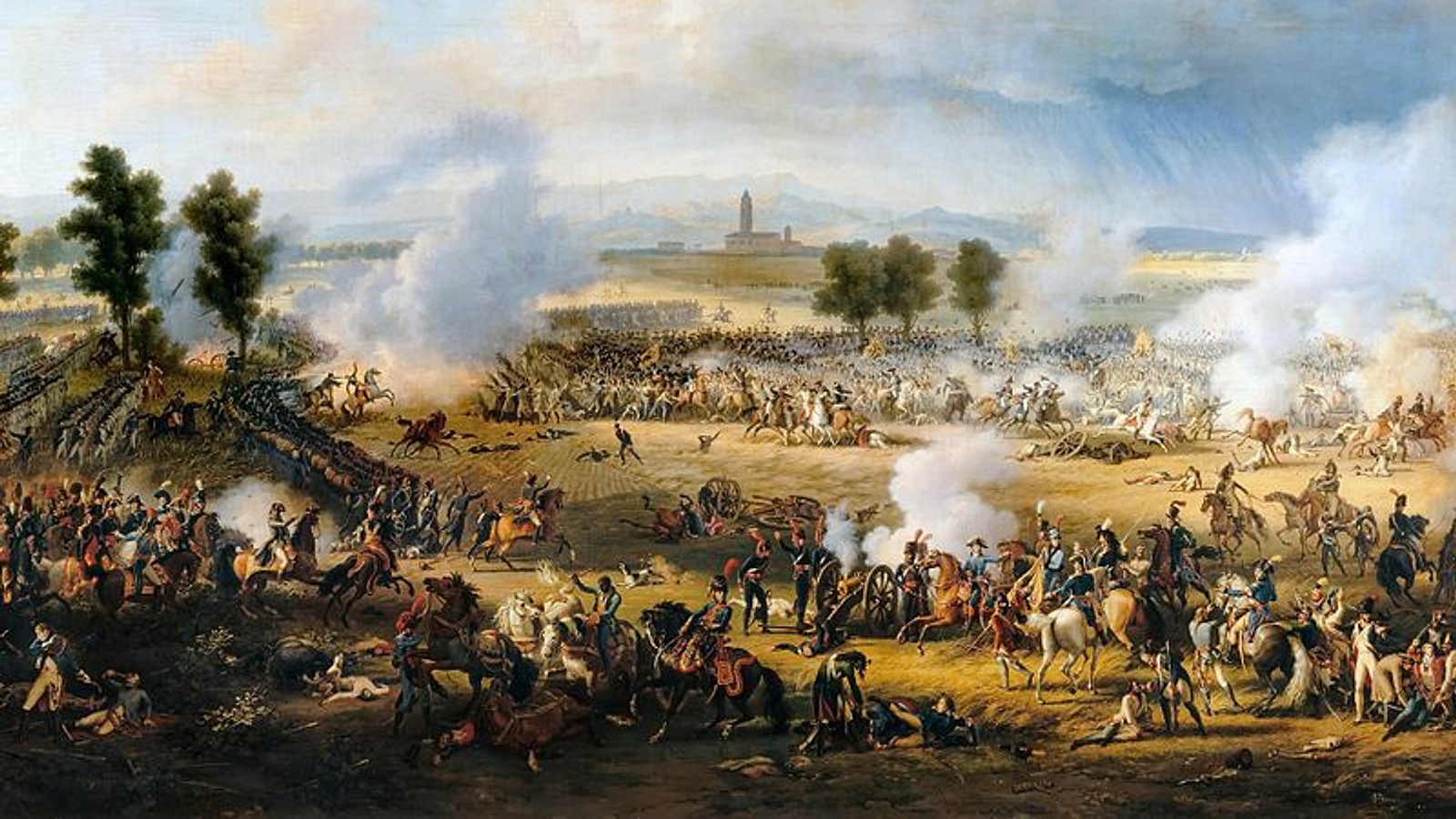The image is a detailed, artistic rendering of an old-fashioned battle scene, capturing the chaos and intensity of war. In the foreground, a wide yellow and green field is populated with dozens, if not hundreds, of men on horseback and on foot, all engaged in fierce combat amidst clouds of smoke. The field is dotted with trees and a small hill to the left. The battlefield is strewn with fallen soldiers and horses, and various parts of the field are shrouded in rising smoke, indicating intense fighting in multiple areas. The scene captures the dynamic movement of horses, some without riders, galloping through the field. In the far distance, a town is visible with a prominent spire, possibly of a church or town hall, standing out against a backdrop of faint mountains. The sky above is dominantly cloudy, with patches of white clouds overlaying a blue sky, adding to the dramatic atmosphere of the battle scene.